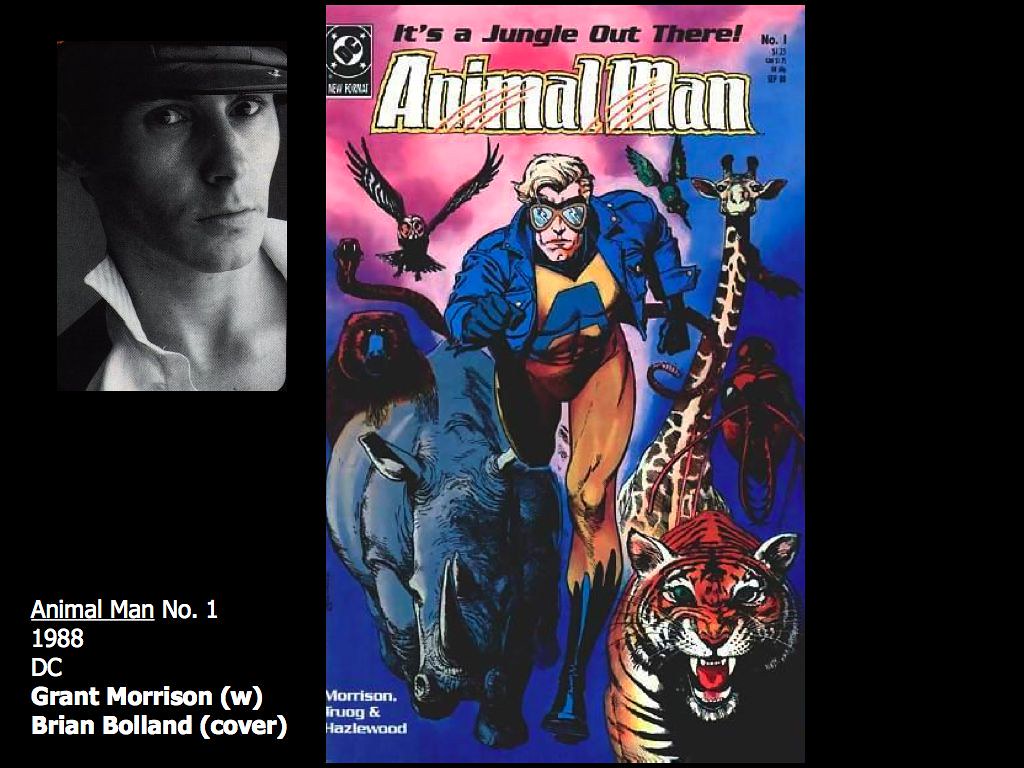This image features two distinct elements: a comic book cover and a black-and-white headshot photo. The comic book cover, prominently positioned in the center, is titled "Animal Man Number 1" from 1988, produced by DC with Grant Morrison as the writer and Brian Bolland as the cover artist. The subtitle reads "It's a Jungle Out There," hinting at the theme. The illustration showcases a serious-looking superhero known as Animal Man, who is depicted running directly towards the viewer. He is adorned in a tight orange leotard, a blue jacket, blackish-blue boots, and goggles over his blonde hair. Surrounding him are a variety of animals, including a tiger, giraffe, rhinoceros, bear, monkey, snake, bird, and more, all vividly colored in hues like gray, orange, yellow, brown, and blue.

To the left of the comic book cover, there is a black-and-white photograph of a man located in the top left corner of the image. This close-up, headshot reveals a clean-shaven man wearing a hat and a white shirt with a black jacket over it. The collar of his shirt is turned up. Below this photo, text reads: "Animal Man, Number 1, 1988, DC, Grant Morrison, W. Brian Bolland, cover."

This detailed description encapsulates elements from all three people's captions and presents a comprehensive view of the image.